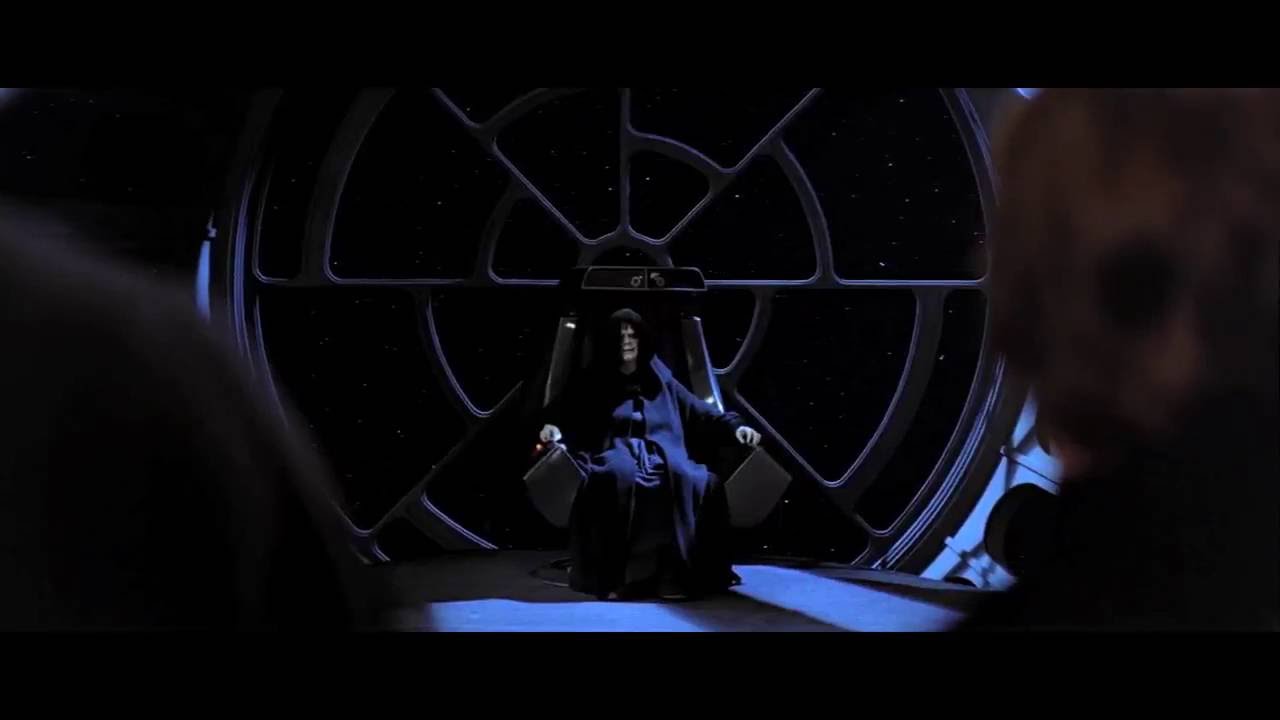This detailed color photograph captures a dramatic scene from a Star Wars movie. In the center of the image, Emperor Palpatine is seated on a black throne, which is positioned in front of a large, round, see-through window showcasing a starry sky, indicating they are in space. Palpatine, shrouded in a long, dark navy blue robe with a hood obscuring part of his face, sits ominously with his hands resting on the armrests of his throne. His skin appears pasty white, adding a menacing aura to his character. The throne is interpreted to have large gray padding on the sides. The room is dimly lit, with the only significant color being a pale blue carpet or mat near the foreground. On either side of the Emperor, two characters stand facing him; their backs are to the camera, revealing only their heads and parts of their cloaks. Though out of focus, one of the characters to the right is suspected to be Luke Skywalker. The silhouettes of other observers in the lower foreground suggest this might be an image capture for the movie, possibly taken during a critical moment on stage or as part of a display.